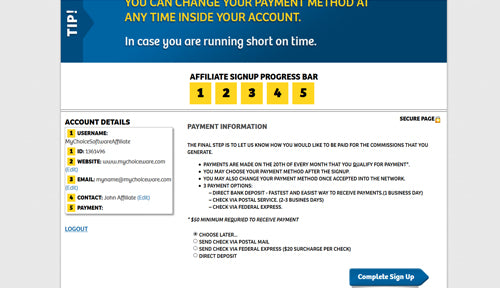The image features a detailed and structured informational interface with several distinct sections and a combination of colorful and monochromatic elements.

The background on the left and right sides is a solid gray color, while the top features a teal background. On the left side of the teal section, there is a bold label "TIP!" in large letters. Just below, in yellow text, it reads: "You can change your payment method at any time inside your account."

Further down, there is a white background with center-aligned text in white that says: "In case you are running short on time." Featured below this text, in black font, is the heading "Affiliate Sign-Up Progress Bar." Below this is a progress bar consisting of five yellow squares numbered 1 to 5 in black, indicating steps from left to right.

On the left-hand side, a black heading reads "Account Details" inside a white rectangular box with a gray outline. Inside this box, each step from the progress bar is detailed in black text next to its respective number. The first step is labeled "Username," the second is blurred and unreadable, the third step is "Website," the fourth is "Email," and the fifth is "Contact," followed by "Payment."

Below this box, an underlined blue text reads "Logout."

A descriptive section titled "Payment Information" follows, detailing the final steps for setting up payment options for the commissions generated. The text mentions that payments are made on the 20th of each month, although part of the text is blurry and hard to read. In this section, the interface provides options to choose the payment method during or after sign-up, although the exact details are somewhat obscured.

At the bottom, the user can select options such as "Choose Later," "Send via Email," "Send a Check via Federal Express," and "Direct Deposit," though some of these options are not entirely legible.